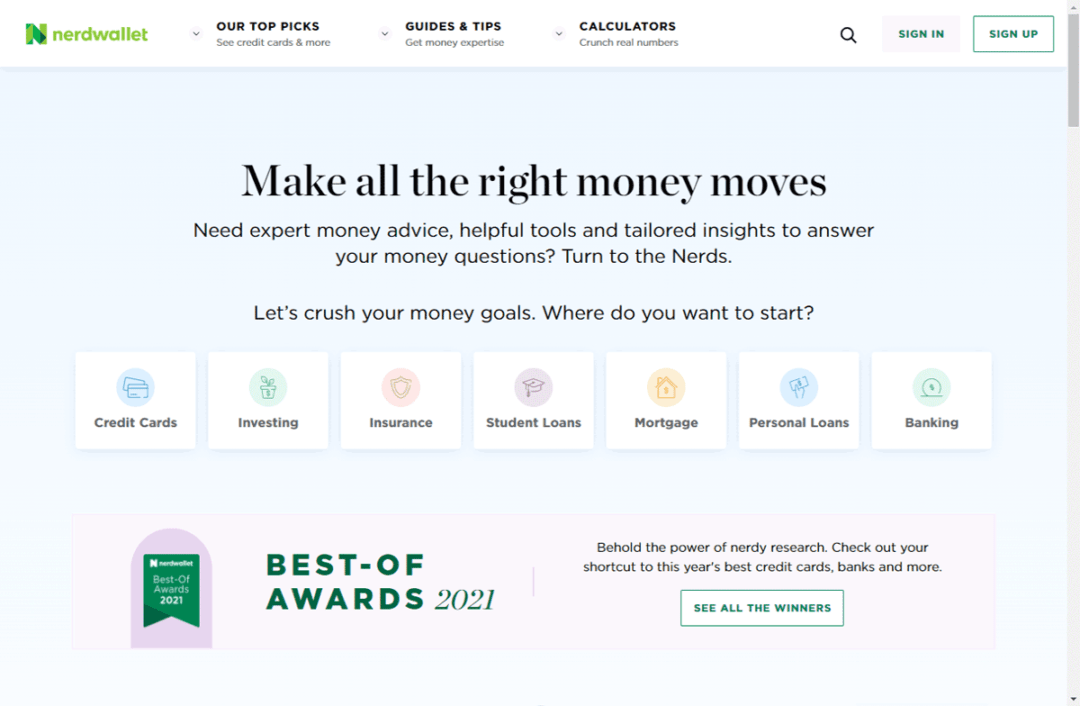This image showcases the landing page of the NerdWallet website, designed in a clean and user-friendly layout. The top left corner prominently features the NerdWallet logo in its signature green color. Adjacent to the logo, several drop-down menus provide easy navigation to various sections: "Our Top Picks," "Credit Cards and More," "Guides and Tips," "Get Money Expertise," and "Calculators, Crunch Real Numbers." Further to the right, users can find a search icon, a sign-in button, and a sign-up button.

Centrally positioned, a bold headline reads, "Make All the Right Money Moves," inviting users to seek expert financial advice, utilize helpful tools, and gain tailored insights to resolve their financial queries with the tagline, "Turn to the Nerds. Let's Crush Your Money Goals. Where Do You Want to Start?" 

Below this call-to-action, various buttons are available, allowing users to quickly access key financial categories such as Credit Cards, Investing, Insurance, Student Loans, Mortgage, Personal Loans, and Banking. At the very bottom of the page, a green "Best of Awards 2021" logo is displayed, highlighting the site’s accolade for excellence.